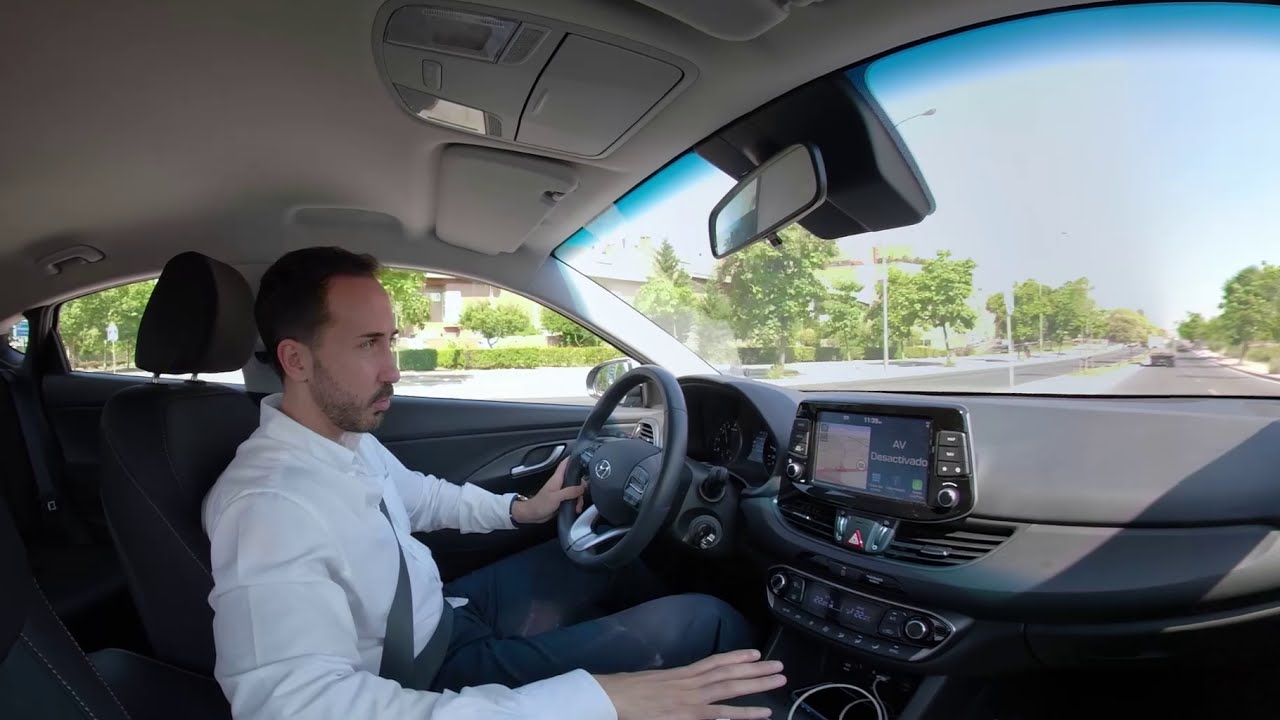The image captures a detailed side view of a man, likely around 35 years of age, driving a modern Subaru. He has closely cropped black hair with a receding hairline and sports a light beard and mustache. Clad in a white, button-down long-sleeve business shirt, he also wears dark gray pants and a gray seat belt. His left hand rests on the steering wheel while his right hand lies casually on his right leg, possibly checking a GPS on the car's dashboard, which is gray. The car's interior blends black seats with a tan headboard. The man is driving through a scenic route surrounded by trees and bushes, under a clear blue sky with no visible clouds. In the distance, a few other cars are visible, indicating he is on a road, perhaps in a neighborhood that features apartment buildings, sidewalks, and light posts. The composition suggests the photo was taken from the perspective of a passenger sitting next to him.